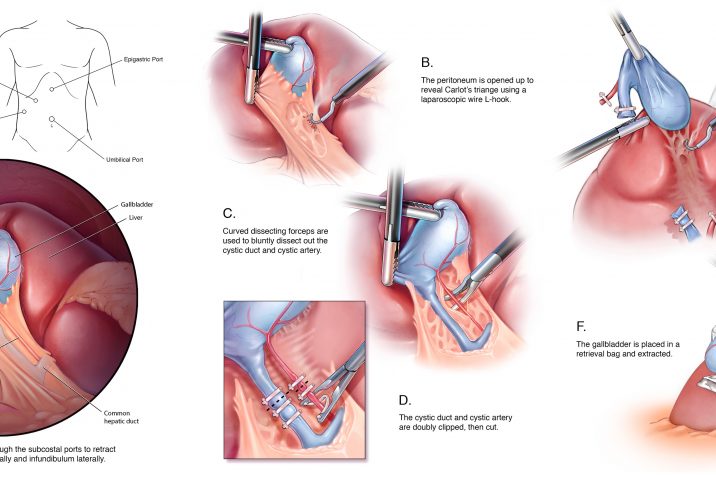The image is a detailed series of illustrations from a medical textbook, specifically depicting the step-by-step process of laparoscopic gallbladder removal surgery. The sequence begins with an outline diagram pointing to a man's abdomen, highlighting anatomical landmarks like the navel. Inset color illustrations show surgical instruments in action.

**Step B**: The periotenium is opened up to reveal Calot's triangle using a laparoscopic wire L-hook device. This step involves careful exposure of the critical structures within the triangle, assisted by the L-hook device, which appears to be cauterizing or dissecting part of the anatomy.

**Step C**: Curved dissecting forceps are employed to bluntly dissect out the cystic duct and cystic artery. The forceps are depicted pulling apart tissues to isolate and expose these ducts.

**Step D**: The cystic duct and cystic artery are doubly clipped and then cut. Illustrations show these structures securely stapled or clipped before being severed to prevent bleeding and ensure safe removal.

**Step F**: The gallbladder is placed in a retrieval bag and extracted from the body. Partial images indicate the use of a retrieval bag for the safe removal of the gallbladder.

The visuals primarily showcase the red and pink hues of the liver and surrounding internal structures, with the cystic duct highlighted in blue and the artery in red for clear identification. The series provides a comprehensive guide to the surgical process, ensuring meticulous instruction for medical professionals.